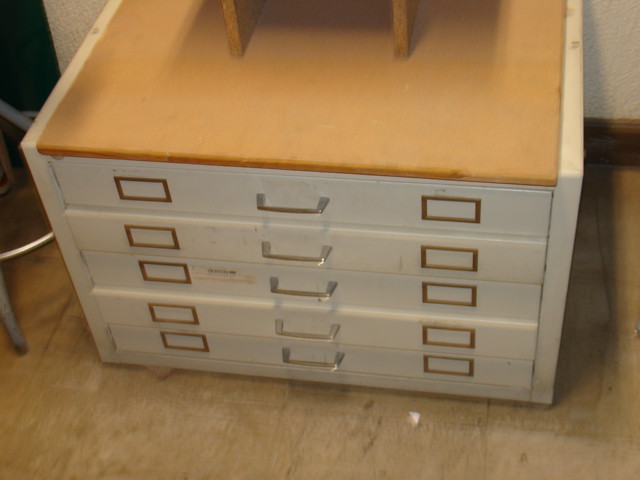This indoor photograph features a white cabinet-like piece of furniture with a butcher block or brown top. The cabinet has five horizontally wide but vertically thin drawers, each adorned with a central silver handle. Flanking each handle are bronze or gold rectangular cardholder frames, totaling ten cardholders. The cabinet rests on a floor that appears to be a grayish-brown plywood with fine grain, reminiscent of a library card catalog. The scene is illuminated by warm indoor incandescent lighting. To the left of the cabinet, the feet and lower structure of a stool with a silver ring and gray legs can be seen. Atop the cabinet, there are two additional wooden slats, though their full form is not visible. The upper corners of the image reveal white stucco walls with dark brown molding at the bottom.